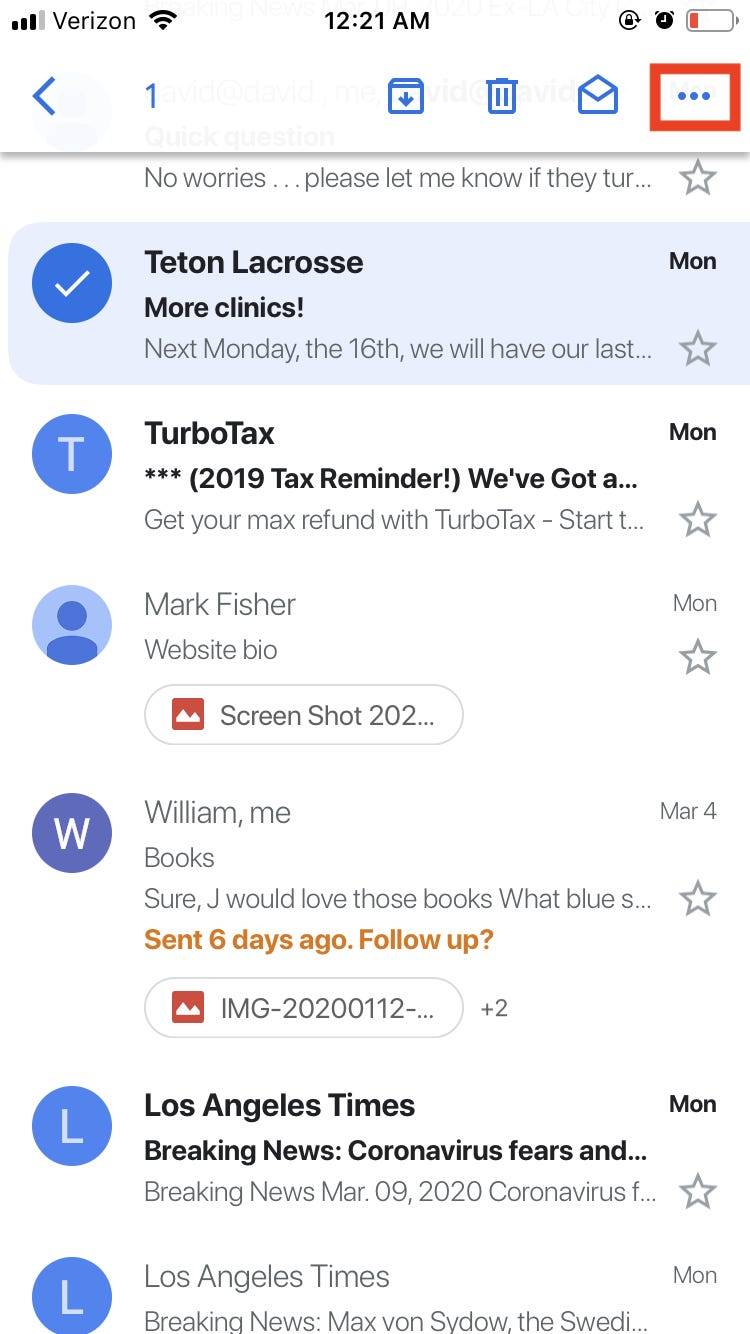The image depicts the Gmail inbox of a user on a mobile device, presumably during nighttime as indicated by the time, 12:21 AM, displayed at the top center of the screen. The user is connected to the Verizon network with visible cell signal and Wi-Fi icons on the top left, while on the top right, there is a screen rotation lock icon, an alarm, and a battery indicator showing a critical low battery level.

Just below the top bar, there is a navigation panel consisting of a back arrow, an archive button, a trash button, a red button highlighted within a red block, and a menu or tab section. 

Within the inbox, several emails are visible. Notably, one email from Turbo Tax is seen. Another email, from Mark Fisher, is noted and it includes a screenshot attachment. An email from William with the subject "Books" is also highlighted, containing two image attachments. Additionally, there are two emails from the Los Angeles Times; one remains unopened and the other has already been read. One of the emails has been selected, indicated by a check mark beside it.